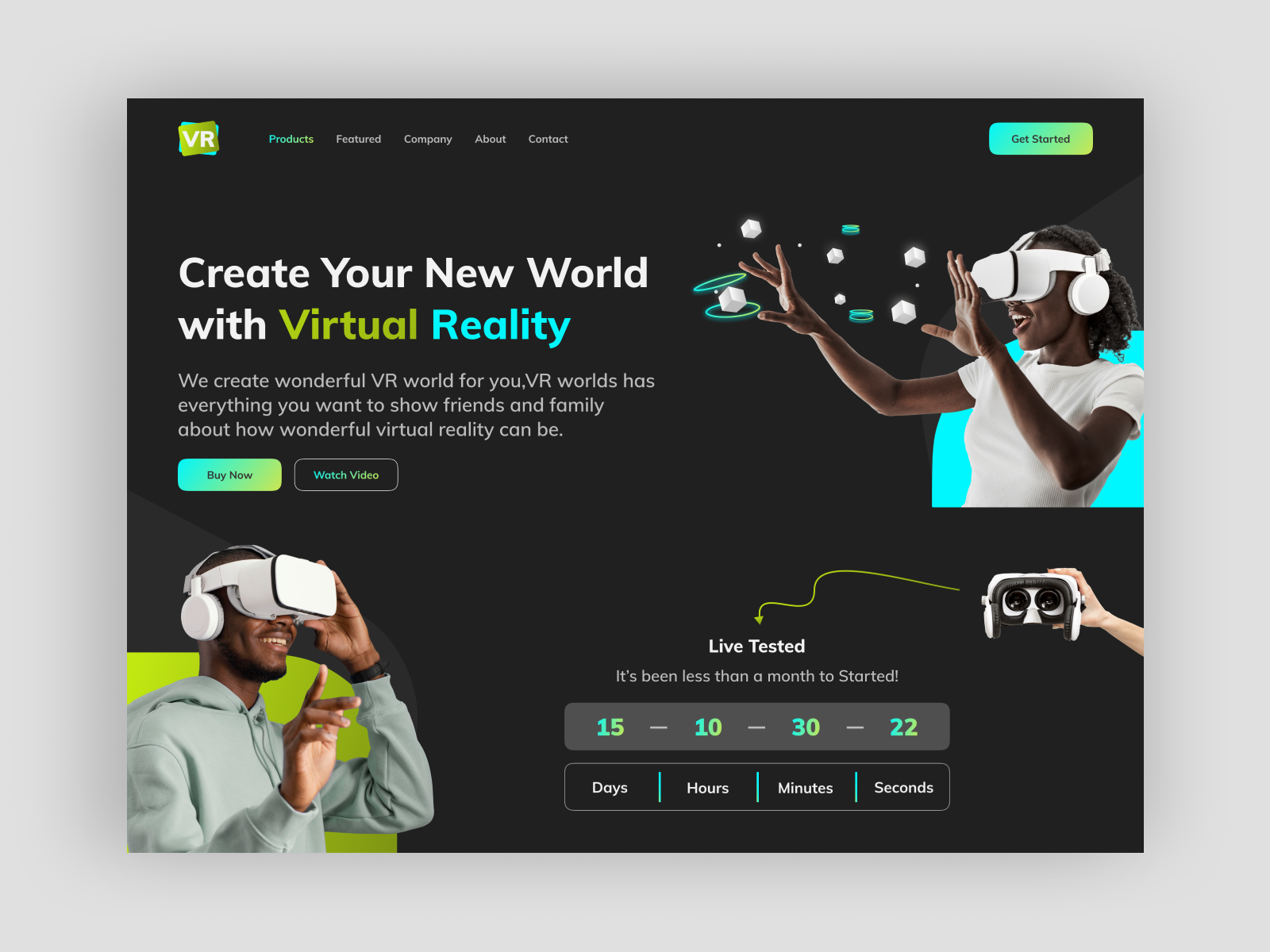The image is a wide rectangular graphic, framed with a thick light gray outline. The central backdrop is predominantly black, split into various interactive sections. 

In the lower left quadrant, a close-up image features a smiling Black man wearing a gray hoodie. He is equipped with white virtual reality headgear and earphones. Behind him, a lime green area accentuates the scene, while his head appears against the black background. The man holds the headgear with his left hand and raises his right hand with fingers extended, gesturing towards the right side of the image.

At the very top of the black background, the capital letters "VR" are displayed in white, with blue and green almost-square sections behind them, seemingly acting as a logo. To the right of this logo, the words "Products," "Featured," "Company," "About," and "Contact" are lined from left to right, with "Products" transitioning from blue to green. The other words remain white, and towards the far right, a "Get Started" button stands out in blue and green with black text.

Above the man's head in the upper left quadrant, a block of text reads:

- "Create Your New World" (in white),
- "With Virtual Reality" (with "Virtual" in green and "Reality" in Tiffany blue),

Three more lines follow beneath:
- "We create wonderful VR worlds for you."
- "VR worlds have everything you want to show friends and family."
- "Learn about how wonderful virtual reality can be."

These lines are in white and contrast with the black background. Below this block of text, a blue-to-green gradient button displays "Buy Now" in black, with rounded corners. Beside it, another button reads "Watch Video" in blue and green, framed by a gray rounded rectangle.

In the upper right quadrant, a smiling Black woman, also wearing virtual reality headgear, faces left. She stands against a Tiffany blue backdrop, wearing a white T-shirt, and extends her arms before her, with fingers splayed. Scattered blue and green circles and cubes float near her, suggesting an interactive VR experience.

The lower right quadrant features an image of a right hand reaching from the right side, holding VR headgear aimed towards the viewer. Nearby, a green squiggly arrow points downwards, accompanied by the text "Live Tested" in white. Below it, a note in light gray reads: "It's been less than a month to start it!"

At the very bottom, a gray bar with rounded edges lists a countdown timer: 

- "15 days," 
- "10 hours,"
- "30 minutes,"
- "22 seconds,"

with "days," "hours," "minutes," and "seconds" in white beneath their respective numbers. The first digit of each time unit is in blue, and the second is in green, separated by blue vertical bars.

Intricate and inviting, the composite image effectively showcases the immersive experience and offerings of virtual reality technology.